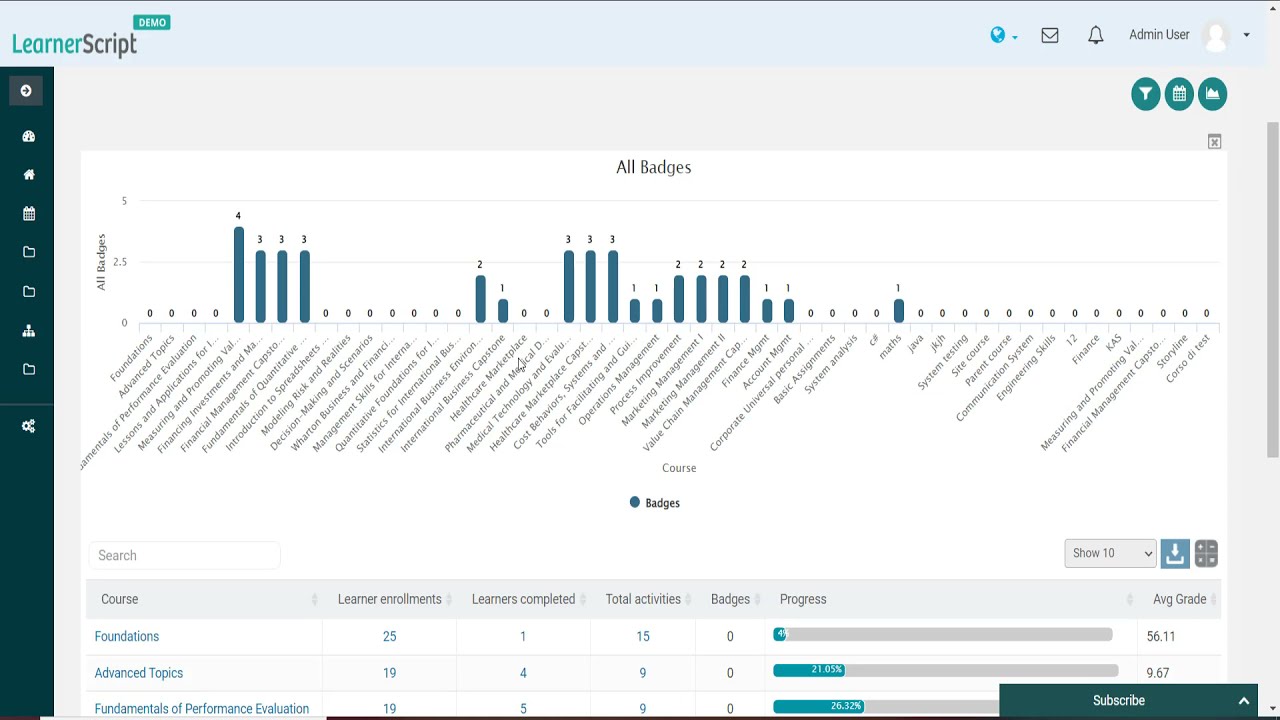This image is a digital screenshot showcasing an instructional dashboard for a training or educational program, likely part of a demo software named "LearnerScript." The interface features a dark blue sidebar menu with icons, including a calendar, visible from the left-hand side. At the top left, the title "LearnerScript" is displayed in light blue aqua and black font, with the word "demo" in a rectangle above the letter T. 

The dashboard is segmented into various sections, with prominent categories such as "course," "foundations," "advanced topics," "fundamentals of performance evaluation," "learner enrollments," "learners completed," "total activities," "badges," "progress," and "average grade." In the middle of the screen, there's a notable header labeled "All Badges," beneath which a bar chart displays different metrics.

The bar chart runs diagonally and lists topics like "foundations," "advanced topics," "fundamentals of performance evaluation," "lessons and applications," "measuring and promoting," "financing investments," "financial management capstone," "introduction to spreadsheets," "modeling risk and realities," "decision making and scenarios," "Wharton business and financials," and "management skills." Each topic is accompanied by blue horizontal bars quantifying statistics, with values ranging from zero to four. Below the chart, statistics related to learner progress are presented, including learner enrollments, completion rates, total activities, and badges earned. 

The top-right corner of the screen includes user interface elements like a bell icon, an envelope sign, and a blank profile picture labeled "admin user." Additional blue circular icons, possibly depicting features like the calendar, are displayed underneath. The layout and data visualization aim to provide a comprehensive overview of educational program performance and participation statistics, making the interface both informative and user-friendly.